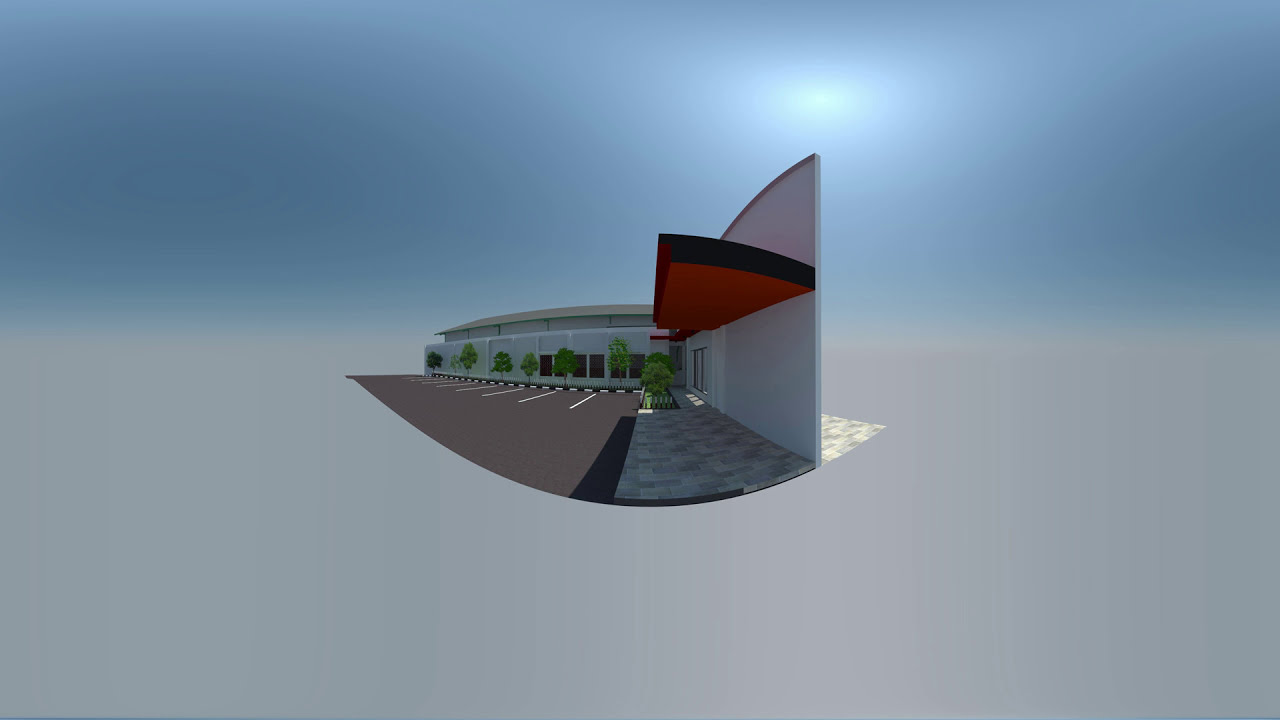This computer-generated image depicts the front elevation of a modern building, appearing to be part of an outdoor shopping center. The building features a prominent white wall with six window panels on the left side and two on the right. A standout characteristic is the red awning that juts out from the right side above the entry door. The ground in front of the building is covered with gray and beige pavers, part of which is cast in shadow. Eight green trees line the entryway, adding a touch of nature to the scene. Adjacent to the building is a parking area on the left side with eight marked spaces for vehicles, distinguished by white lines on the dark gray asphalt. The background of the image transitions from a steely blue at the top to light gray at the bottom, giving the impression that the design is suspended in space.